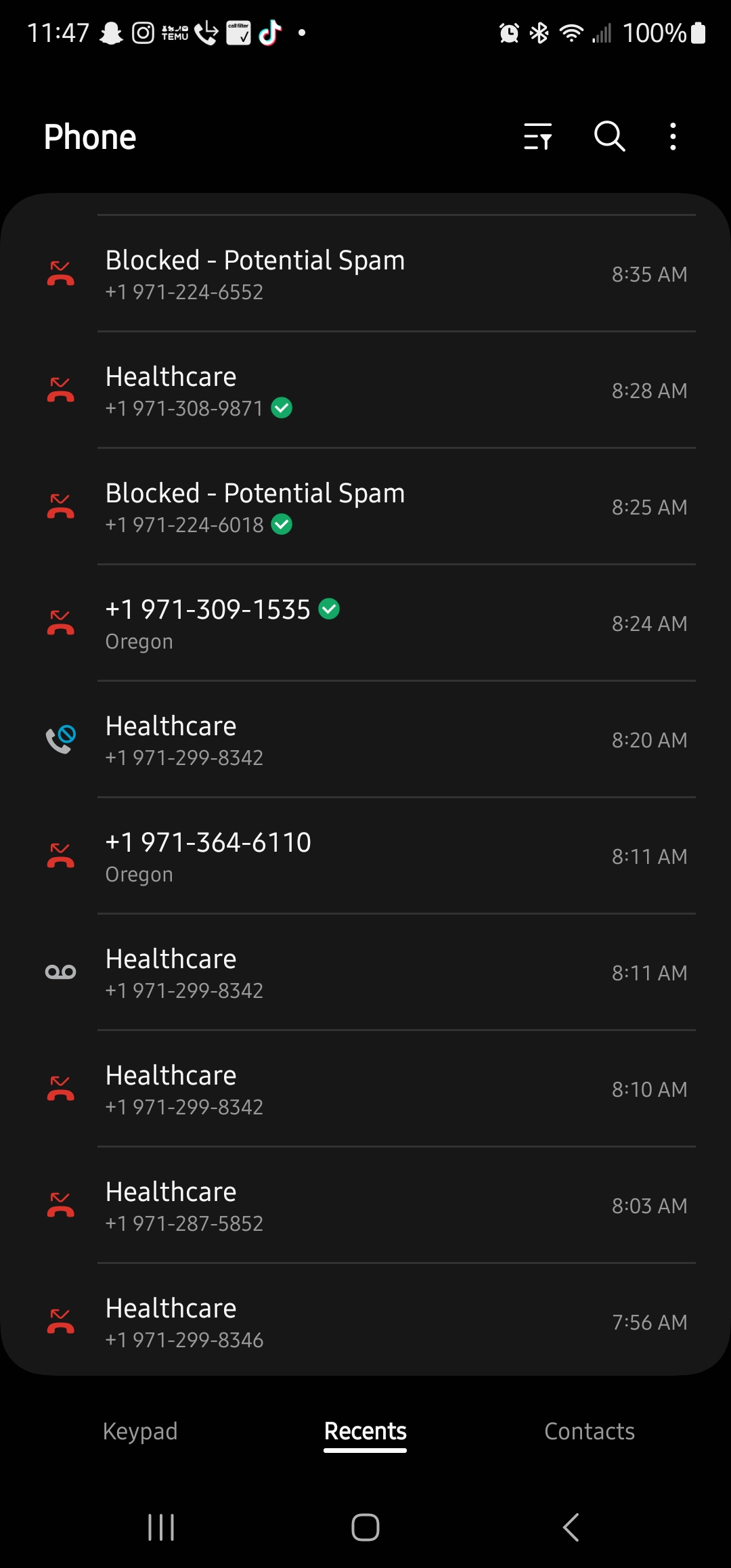A screenshot of a recent call log on a smartphone, displayed in dark mode with a black background and white text, reveals a series of incoming calls. Many of the calls are marked as either missed or blocked. The icons next to each entry help identify the nature of the calls. The first entry is labeled "Blocked - Potential Spam," followed by "Healthcare," another "Blocked - Potential Spam," "Missed Call" from a number starting with 971, several "Healthcare" entries, and finally, a voicemail left under the "Healthcare" label. The calls were received in quick succession within a 40-minute period, starting at 7:56 AM and ending at 8:35 AM. This pattern suggests the individual is experiencing a high volume of spam calls, with some managing to bypass block filters, possibly through call spoofing techniques that the phone's software fails to recognize consistently.